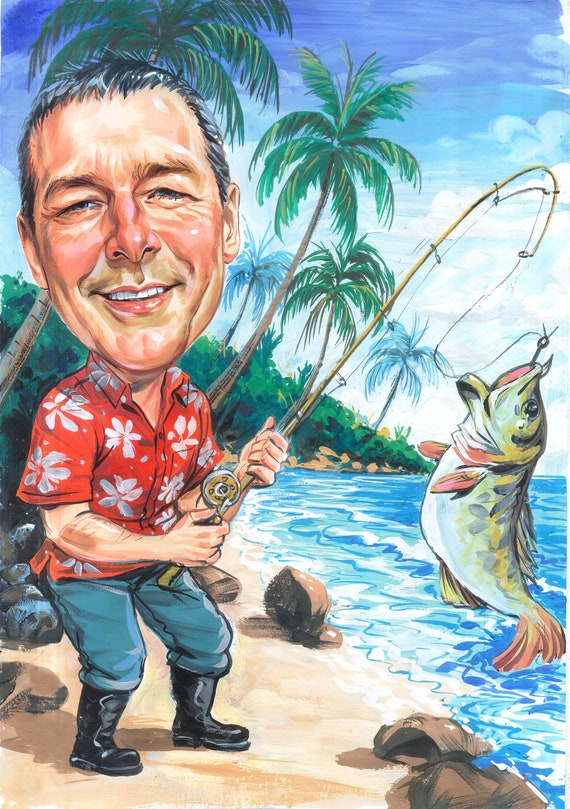The image is a cartoonish caricature of a comical-looking white man on a small sandy beach. He has disproportionate body parts, with an oversized head that's about as large as the rest of his body. The man has short black hair, pink cheeks, a pink nose, and is smiling broadly with squinty eyes, showcasing his very white teeth. He appears slightly sunburned and sports a red Hawaiian shirt with white blossoms, dark blue jeans tucked into black boots. 

In his hands, he holds a bamboo fly fishing rod with a large, colorful fish hooked by its lip. The fish, about three-quarters the size of the man's body, has a cartoonish appearance with greenish, black, and blue hues, and pinkish tail and fins.

The backdrop reveals a vibrant blue ocean with gentle waves lapping at the white sandy shore, dotted by a few brown rocks casting shadows. Behind him, a lush forest with palm trees leaning over the water and a vegetation-covered hillside slopes down towards the sea. The sky is mostly blue with hints of overcast, providing a serene yet whimsical setting for this exaggerated scene.